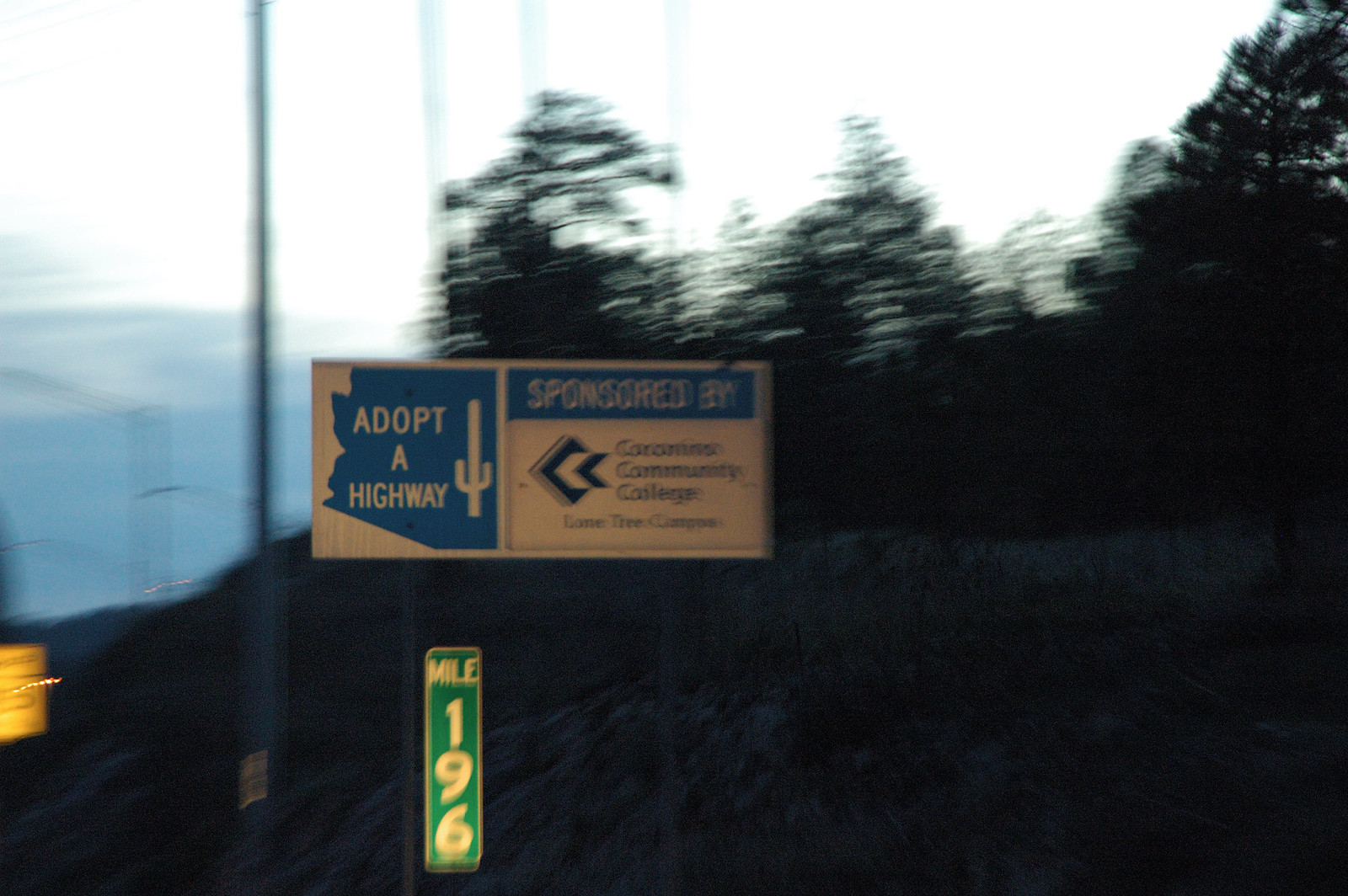The photograph captures a moment taken by a driver currently on the road, evidenced by the motion blur that accompanies the image. The scene is set on an upward stretch of the road, bordered by trees on the right side, which stand atop a hill of dirt. On the left side of the image, two road signs come into view. One is a partially obscured yellow sign that resembles a speed limit indication, displaying a discernible "5" but with the remaining digit illegible. Prominently positioned in the center of the frame is a blue and white "Adopt a Highway" sign, sponsored by a community college, though the blurred text beneath remains unreadable. Below it stands a green mile marker sign, indicating Mile 196, with the mile number arranged vertically and the word “mile” horizontally.

Further road infrastructure features include tall metal poles, likely road lights, adding to the highway’s structure. The backdrop reveals that the photo was taken either at sunset or sunrise, with the sky transitioning from light to dark—a gradient of light hues at the top of the sky to a deeper dark blue on the left side, suggesting the mixing of day and night.